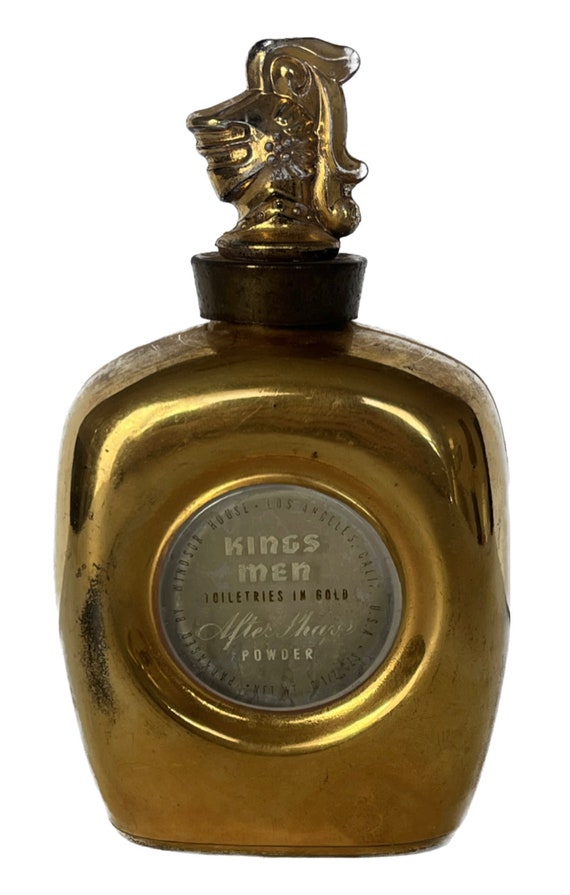This is a photograph featuring an antique, gold-colored bottle set against a white background. The bottle, which could be an aftershave powder container, bears the words "King's Men" and "Toiletries" prominently within a gray circular label on its front. The label also includes illegible smaller text around the circle. The bottle's capped with a detailed topper resembling a knight’s helmet, complete with a front mask and what appears to be a plume of feathers extending outward. The helmet is brushed brass or gold, matching the bottle's well-worn exterior, which shows signs of wear with white edges and blackening on one side. The bottle has visible indentations and pitting, which, along with reflections, emphasize its antique nature.